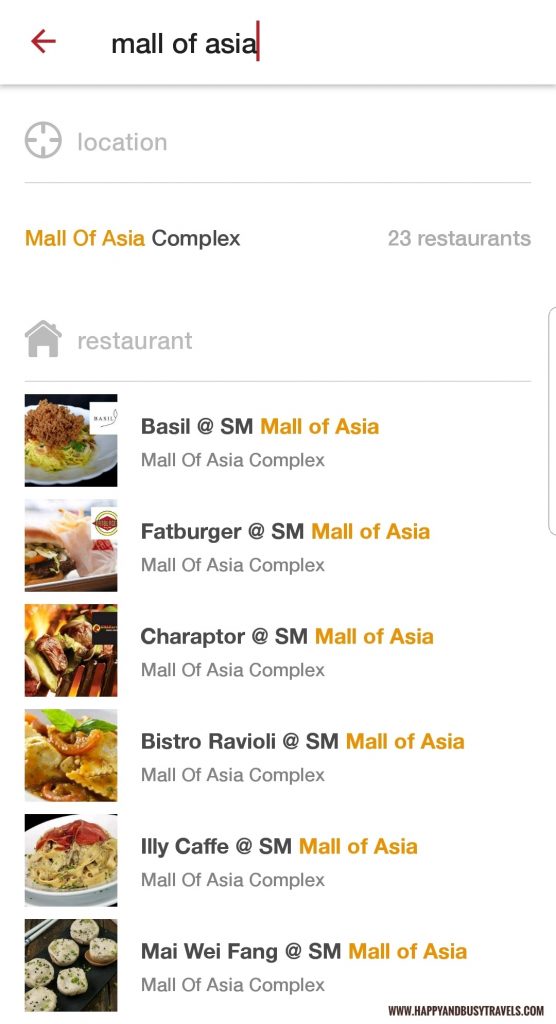This image is a screenshot, likely taken from a smartphone, of a web page from the website HappyBusyTravels.com. The web page features a list of restaurants located in the Mall of Asia. "Mall of Asia" is prominently highlighted in yellow, while the rest of the text is in black and grey. Below the restaurant listings, there are various food options mentioned, including items such as a fat burger, ravioli, and basil. According to the web page, there are a total of 23 restaurants available at the Mall of Asia.